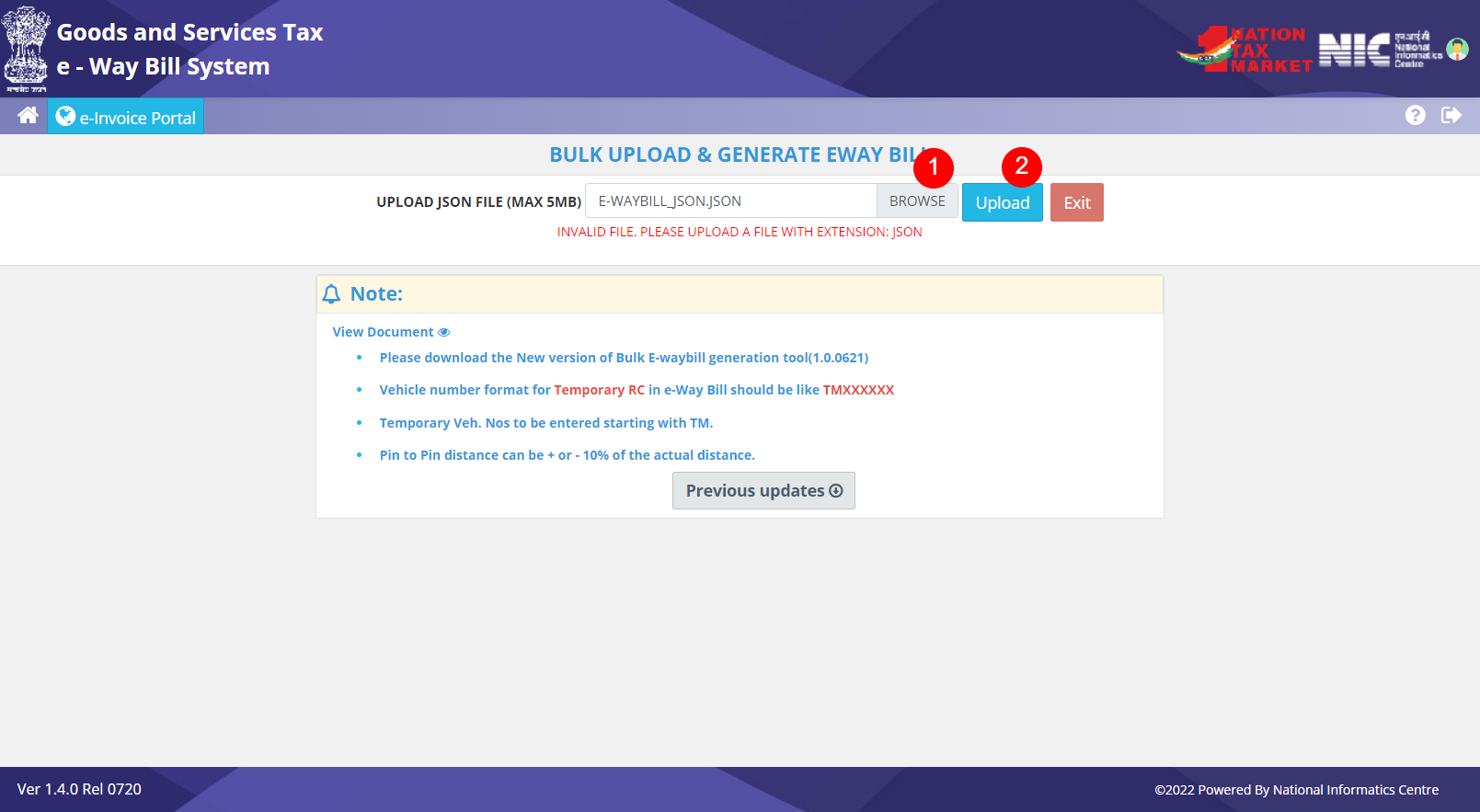The image is a detailed screenshot of a website dedicated to the Goods and Services Tax (GST) e-Way Bill System. The top header features a gradient border transitioning from dark purple to light purple. In the upper left corner, "Goods and Services Tax e-Way Bill System" is displayed in white text. To the right, there are three distinct elements: a logo with a large red number "1" accompanied by the text "Nation Tax Market," an "NIC" logo with some smaller text beneath it, and an avatar picturing a male figure on a green background.

Below this header is a lighter blue border serving as a navigation bar. On the left, there's a home icon representing the homepage. Next to it, a turquoise button with a globe icon labeled "e-Invoice Portal" is prominently visible. On the right side of this bar, there is a white circle icon containing a question mark and a right arrow, followed by blue text reading "Bulk Upload and Generate e-Way Bills."

Beneath this navigation bar lies the main interactive section of the page. On the left, instructions to "Upload JSON File (max 5mb)" are displayed next to a search box. To the right are three buttons: a gray "Browse" button, a blue "Upload" button, and a reddish-brown "Exit" button with "EXIT" written in white. Small red circles with numbers "1" and "2" are overlaid on the "Browse" and "Upload" buttons, respectively. Below this section, a red text alert states, "Invalid file. Please upload a file with extension JSON."

Further down, a prominent notice box is outlined with a yellow border at the top, featuring a bell icon and the word "Note." Inside, the box has a white background with blue text that reads "View Document," followed by four bullet points:
1. "Please download the new version of Bulk E-Way Bill Generation Tool."
2. "Vehicle number format for temporary RC and E-Way Bill should be like TMXXXXXX."
3. "Temporary VEH NOS to be entered starting with TM."
4. "Pin to pin distance can be plus or minus 10% of the actual distance."

A grey button labeled "Previous Updates" resides at the bottom of this notice box.

At the bottom of the page, another border matches the design of the top header, featuring a dark purple to light purple gradient. On the left side, white text reads "VER 1.4.0-REL-0720," while on the right side, a copyright notice informs users: "© 2022 Powered by National Informatics Center."